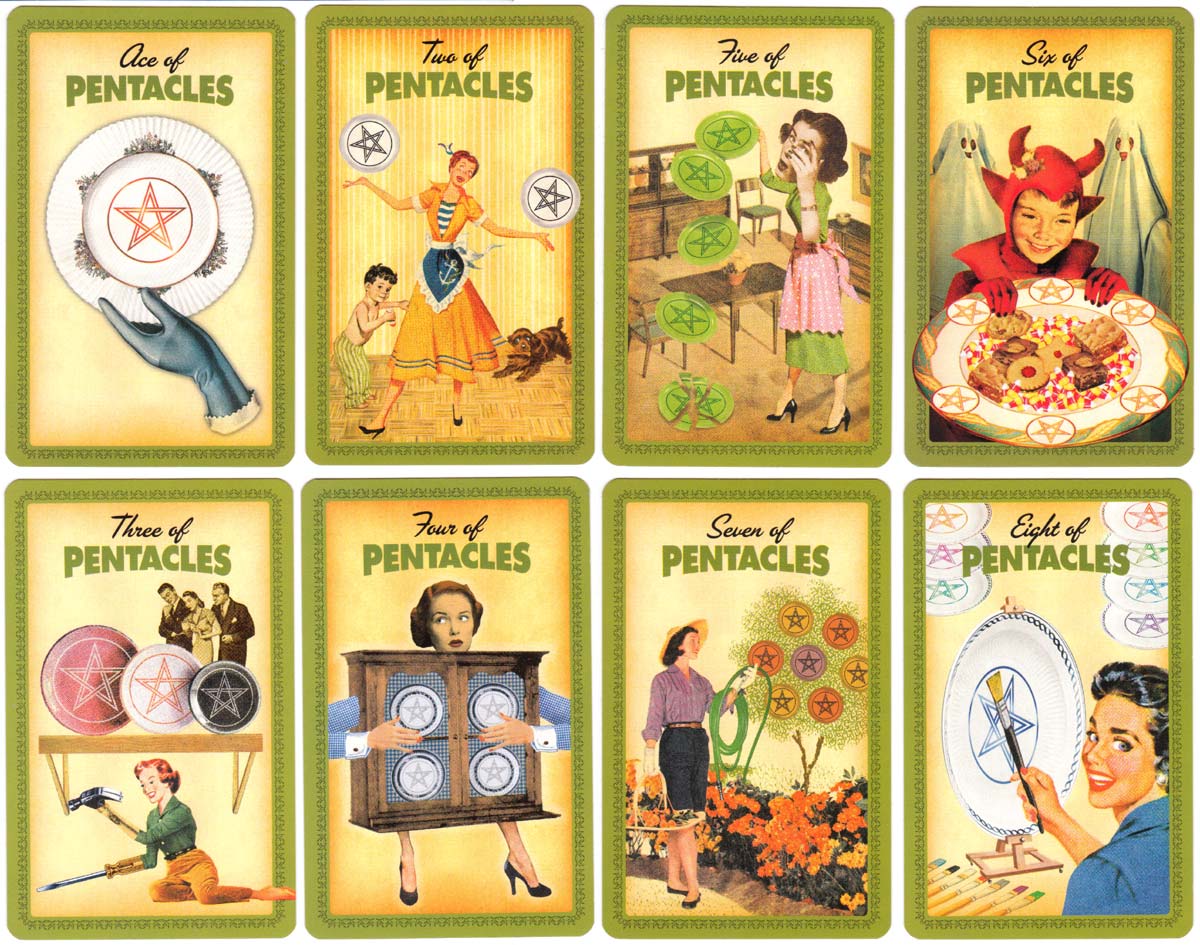This image features a set of eight tarot cards arranged in a neat grid of two rows, each containing four cards. Each card is bordered by a green frame and has a generally yellow background. The text at the top of each card reads, in order from the top left to the last card: Ace of Pentacles, 2 of Pentacles, 5 of Pentacles, 6 of Pentacles, 8 of Pentacles, 7 of Pentacles, 4 of Pentacles, and 3 of Pentacles. The illustrations on the cards are old-fashioned, evoking 1950s and 1960s aesthetics, each depicting different figures engaging in various actions. For example, the 6 of Pentacles card shows a boy in a red devil costume looking over a plate of desserts, while the Ace of Pentacles card depicts another figure. Each card also features a 5-pointed star, and the figures appear to interact with these stars in different ways. The overall style of the image has a quirky blend of retro fashion and mystical elements.